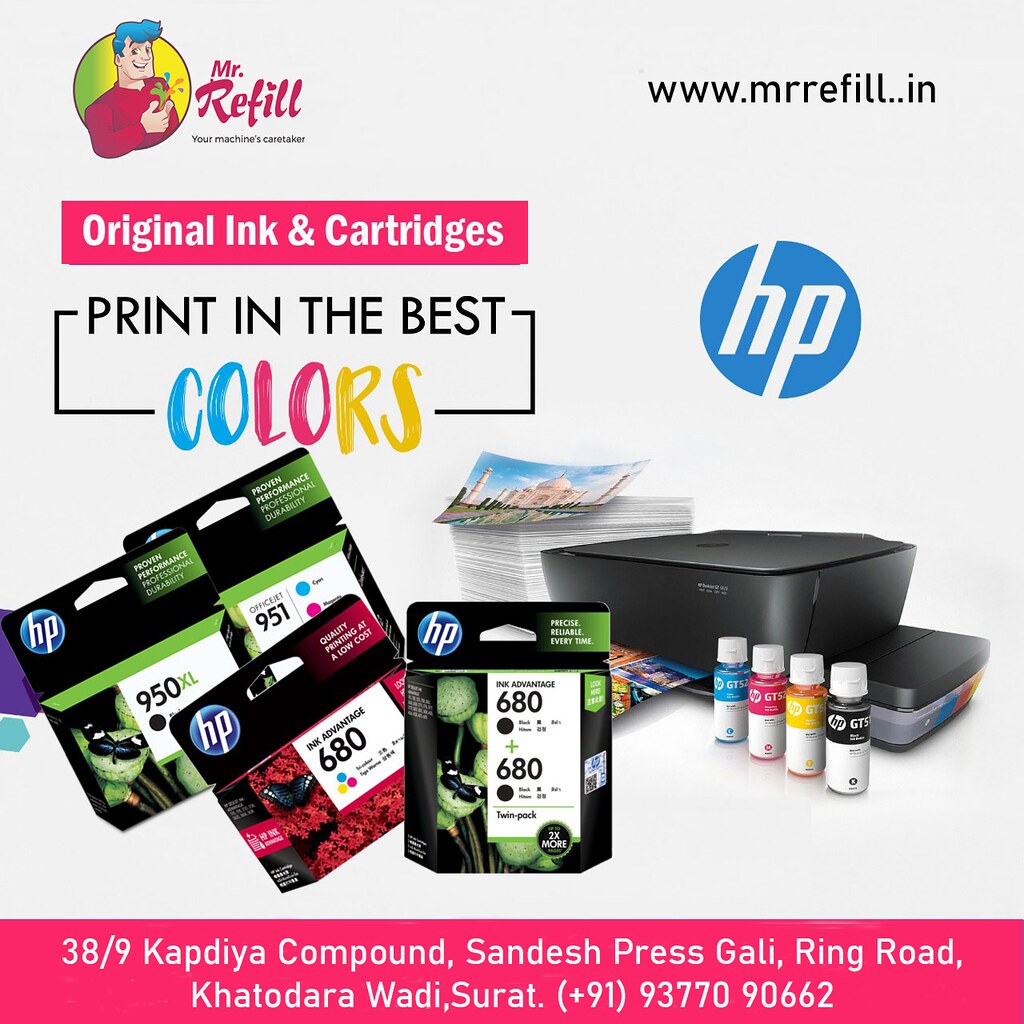This square-shaped advertisement for HB and HP ink cartridges features a white background prominently displaying the Mr. Refill branding. In the upper left corner, there is a cheerful cartoon of a man with blue hair and a red shirt, adjacent to the text "Mr. Refill" and the website www.mr.refill.ink. The tagline "Original ink and cartridges print in the best colors" is highlighted, emphasizing the quality of the prints produced. To the right, the blue and white HP logo is visible, accompanied by images of various HP ink cartridges, including models 950XL, 951, and 680. Beneath these elements, a Hewlett Packard printer is showcased with vibrant photographs emerging from it, underscored by four refill bottles in black, yellow, magenta, and cyan. The bottom of the image features a vivid pink bar containing detailed contact information: "38/9 Cappy dia compound, Sandesh Press Gali, Ring Road, Katodara Wadi, Surat," along with a phone number for inquiries, "+91 93770 90662."